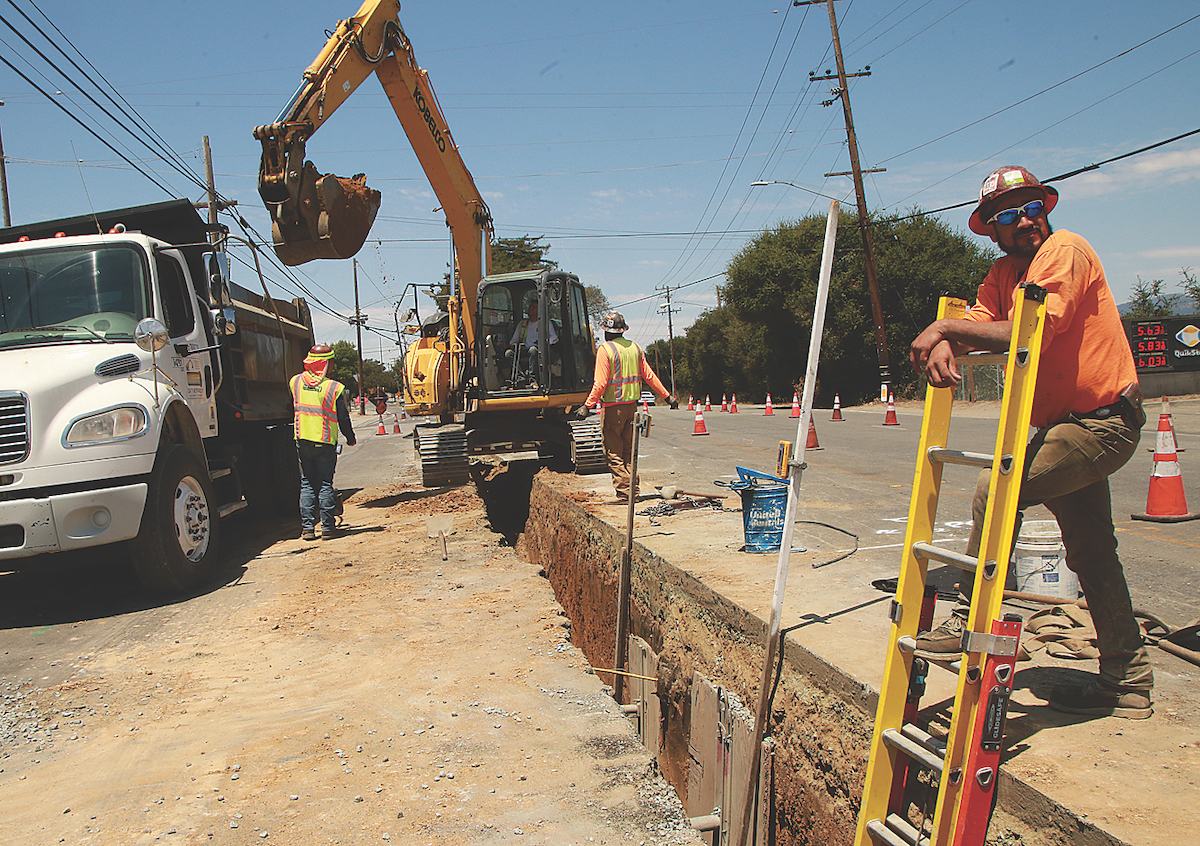This rectangular photograph vividly captures a roadside construction scene under a clear, blue sky punctuated by some power lines in the distance. The setting spans a transition from a dirt ground to a paved concrete road, partially blocked off by orange and white safety cones. Central to the image is a piece of heavy yellow construction equipment with a crane arm extending over the bed of a large white dump truck with a black bin on the back. 

In the foreground, a small concrete barrier runs parallel to the crane, atop which stand two construction workers. One worker, wearing an orange shirt, brown pants, brown work boots, and sunglasses, leans against a yellow ladder. His crossed arms and commanding stance face the camera, giving a clear view of his attire and expression. The other worker, clad in a yellow safety vest and hard hat, is positioned behind him, walking towards the crane. Further back, another worker in a yellow vest and hard hat operates the heavy equipment, though his details are obscured due to distance.

The image showcases the meticulous process of trench digging, as indicated by the ladder that descends into the trench and the presence of both dirt and paved sections of the road. This bustling scene is framed by additional safety measures, including reflective cones and work attire, underscoring the organized labor taking place in what seems to be a suburban neighborhood. Nearby trees and cables add further context to this dynamic and detailed construction view.